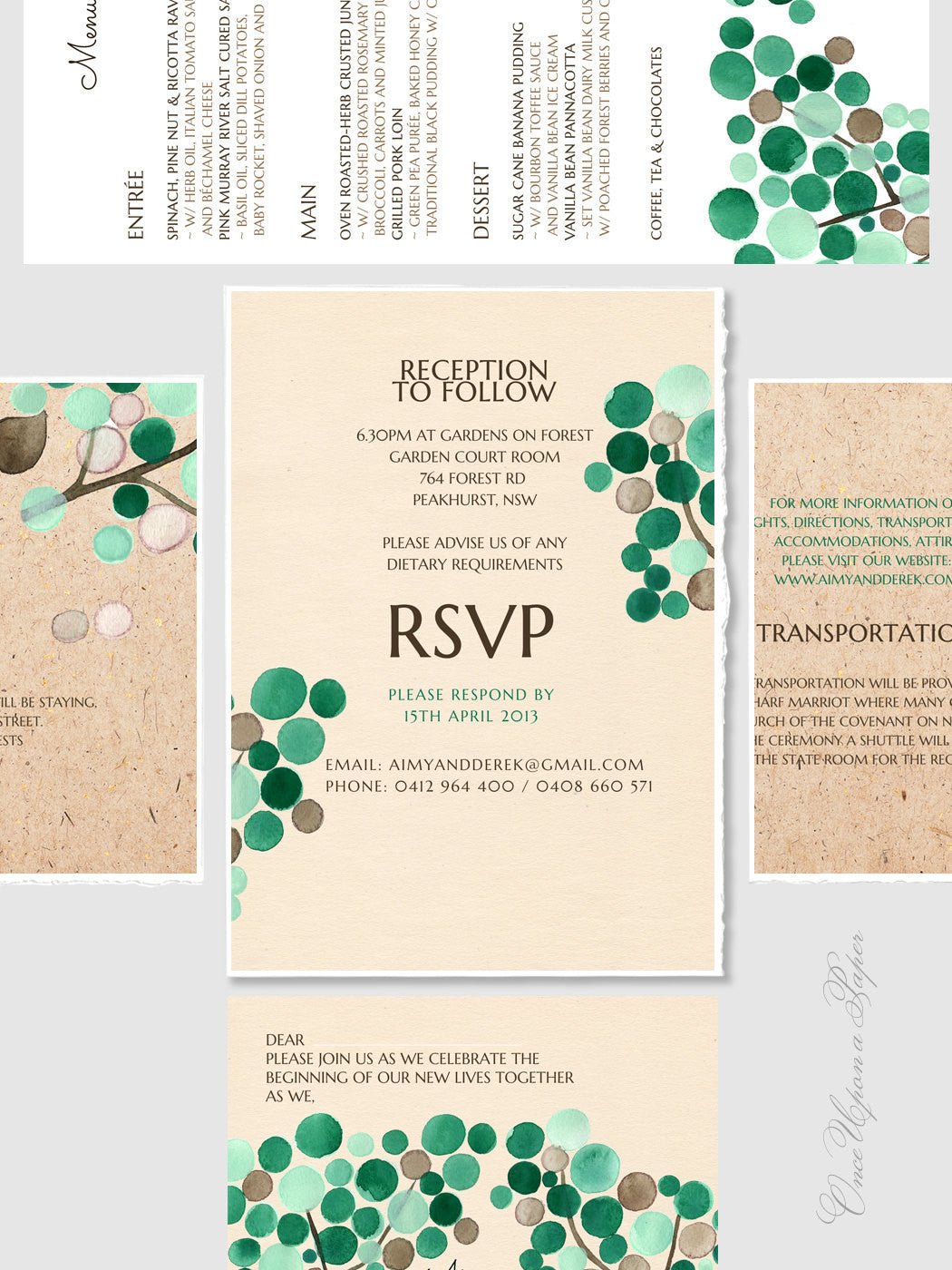The image features an elegant invite for a wedding celebration. The central pamphlet has a beige background adorned with green, light green, dark green, and mint green dots resembling buds attached to a stem. In brown text, it announces, "Reception to follow, 6:30 PM at Gardens on Forest, Garden Courtroom, 764 Forest Road, Peakhurst, NSW." It also requests recipients to "Please advise us of any dietary requirements." Below, in capitalized text, it states, "RSVP," followed by instructions to respond by 15th April 2013, with contact information: email amyandderrick@gmail.com, phone numbers 0412-964-400 and 0408-660-571. At the bottom, partially visible is the wedding invitation itself, starting with "Dear," and an invitation to "Please join us as we celebrate the beginning of our new lives together." Decorative accents of green dots on stems are consistent throughout the text. At the top of the image, there is a sideways menu detailing the entrees, main dishes, and desserts to be served.